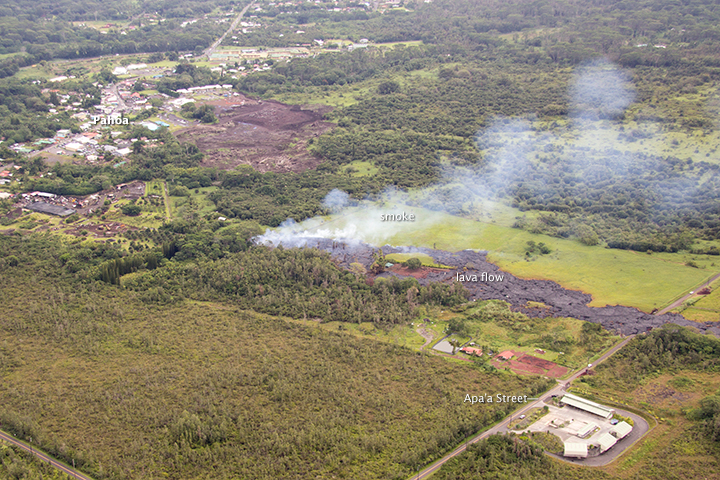The aerial photograph depicts a vibrant, natural landscape with an intricate mix of greenery and human habitation. Dominating the top portion of the image is a dense forest, and this greenery extends towards the middle right side where it intersperses with an expansive grassy area. The image includes clear, labeled captions: "Pahoa" in the top left corner, marking a small town characterized by a few white houses. In the center, the label "Smoke" points to a visible smoke trail emanating from the ground, indicative of volcanic activity. This trail of smoke extends towards the middle right where it converges with a label indicating "Lava Flow." Here, you can distinctly see a stretch of black ash flowing from the smoke area towards the right middle of the picture, cutting across the grassy terrain. Towards the bottom right corner, the image marks "Apa'a Street," suggesting a road potentially compromised by the volcanic flow. The overall setting is illuminated by natural light, adding to the clarity and vividness of the scene.